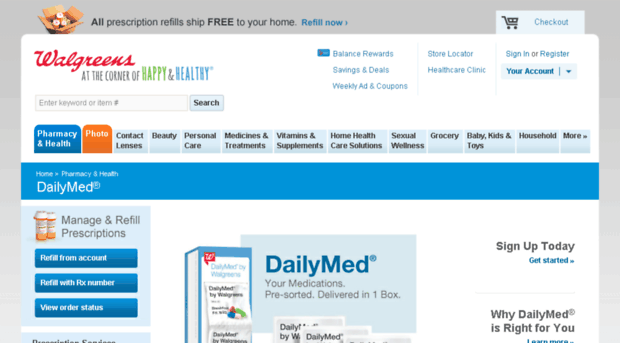Image Description: 

The image features a gray rectangular background with a white rectangular section on top. At the very top of the gray area, there is an open cardboard box containing several prescription bottles. The text within this section reads in black letters, "All prescription refills ship free to your home," followed by "Refill now" in blue letters. Below this is a blue "Checkout" button with a small shopping cart icon.

In the white rectangle, the red Walgreens logo is positioned prominently. To the right of the logo, there are the words "Corner of" in black, "Happy" in white, and "Healthy" in blue. Below this, there is a search button, and adjacent to it are categories listed in blue: "Balance Rewards," "Savings & Deals," "Weekly Ad & Coupons," "Store Locator," "Healthcare Clinic," and "Sign In or Register Your Account."

Underneath this row, there are several small squares and rectangles laid out horizontally, representing different sections of the website. The first category is "Pharmacy & Health" in blue, followed by "Photo" in red. The subsequent categories are in a lighter blue: "Contact Lenses," "Beauty," "Personal Care," "Medicare," "Medicines & Treatment," "Vitamins & Supplements," "Healthcare," "Home Healthcare Solutions," "Sexual Wellness," "Groceries," "Baby," "Kids & Toys," "Households," and "More."

Below, there is a blue rectangle labeled "Daily Meds." Following this is a lighter blue rectangle that states "Manage and Refill Prescriptions." Subsequently, there are two dark blue rectangles: "Refill from Account," "Refill with RX Number," and a third dark blue option for "View Order Status." 

In the middle right section of the image, there is a box containing medicines. Text alongside the box reads: "Daily Med, your medicines, pre-sorted delivery in one box." Below this is a sign-up prompt with "Sign Up" in black and "Get Started" in blue. Additional information follows with "Why Daily Med is right for you" and a clickable "Learn More" in blue, with the rest of the text in black.